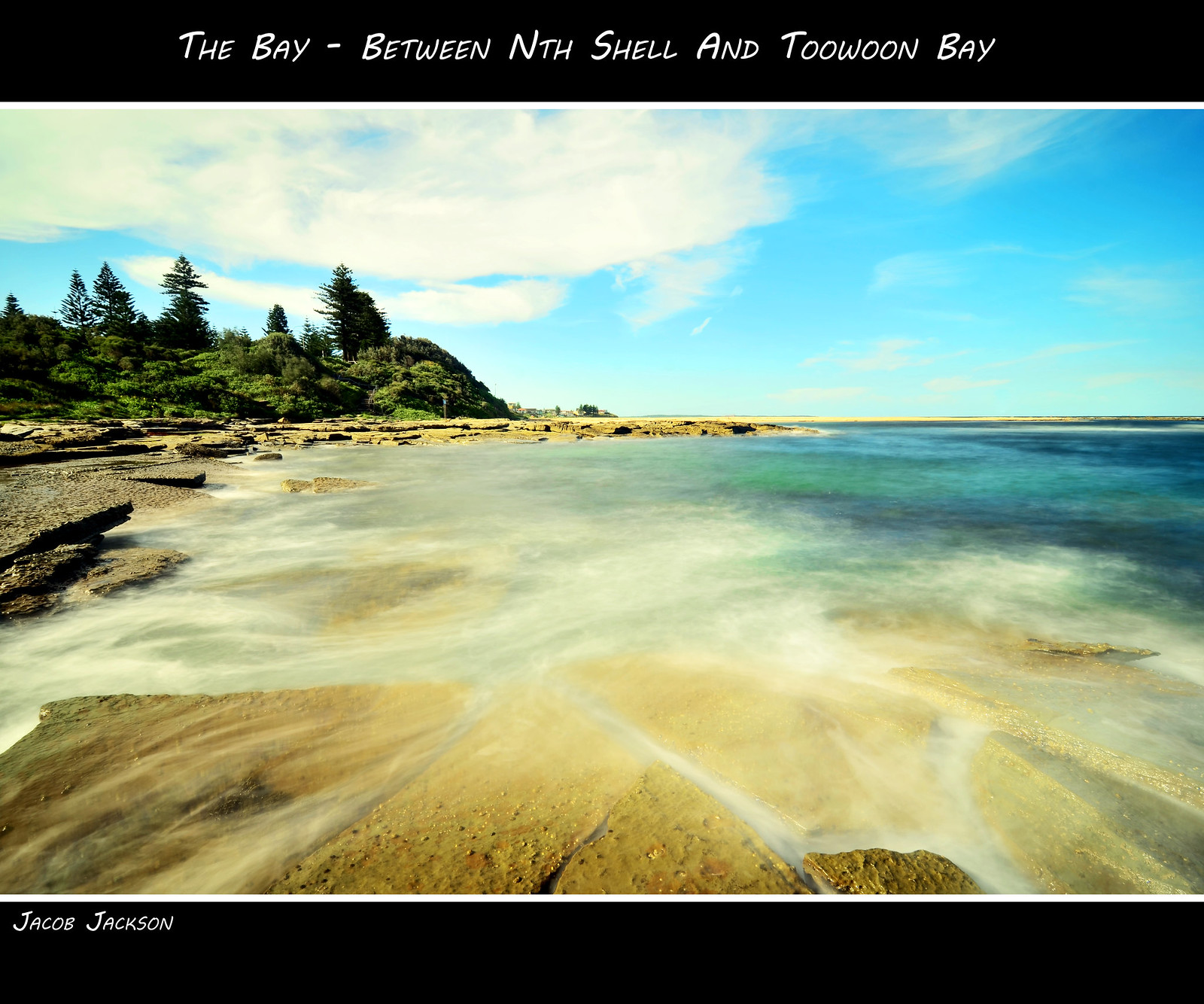The photograph captures a stunning, bright beach scene framed with black borders at the top and bottom, with white text and an additional smaller white border separating the image from these frames. The text at the top reads, "The Bay, between Inchel and Tuon Bay," whereas the bottom text in the left corner reads, "Jacob Jackson."

The scene itself is set against a backdrop of a clear blue sky over the ocean to the right, with the upper left part of the sky adorned with white cumulus clouds, suggesting a sunny morning or early afternoon. The center of the photograph showcases a vibrant beach where the sea washes up onto the shore, framed by a rocky shoreline that winds from the left to the middle of the picture. Between the rocks, there appears to be a captivating mist or sea foam that adds a mystical quality to the scene.

To the left, the rocky shore transitions into verdant green hills covered with bushes and possibly evergreen trees, enhancing the natural beauty of the landscape. In the lower half of the image, the bright sunlight accentuates the fine details of the shore, rocky formations, and the interplay between the mist and water. Overall, the photograph masterfully combines natural elements and text to deliver a vivid, almost picturesque representation of a serene coastal environment between Inchel and Tuon Bay.